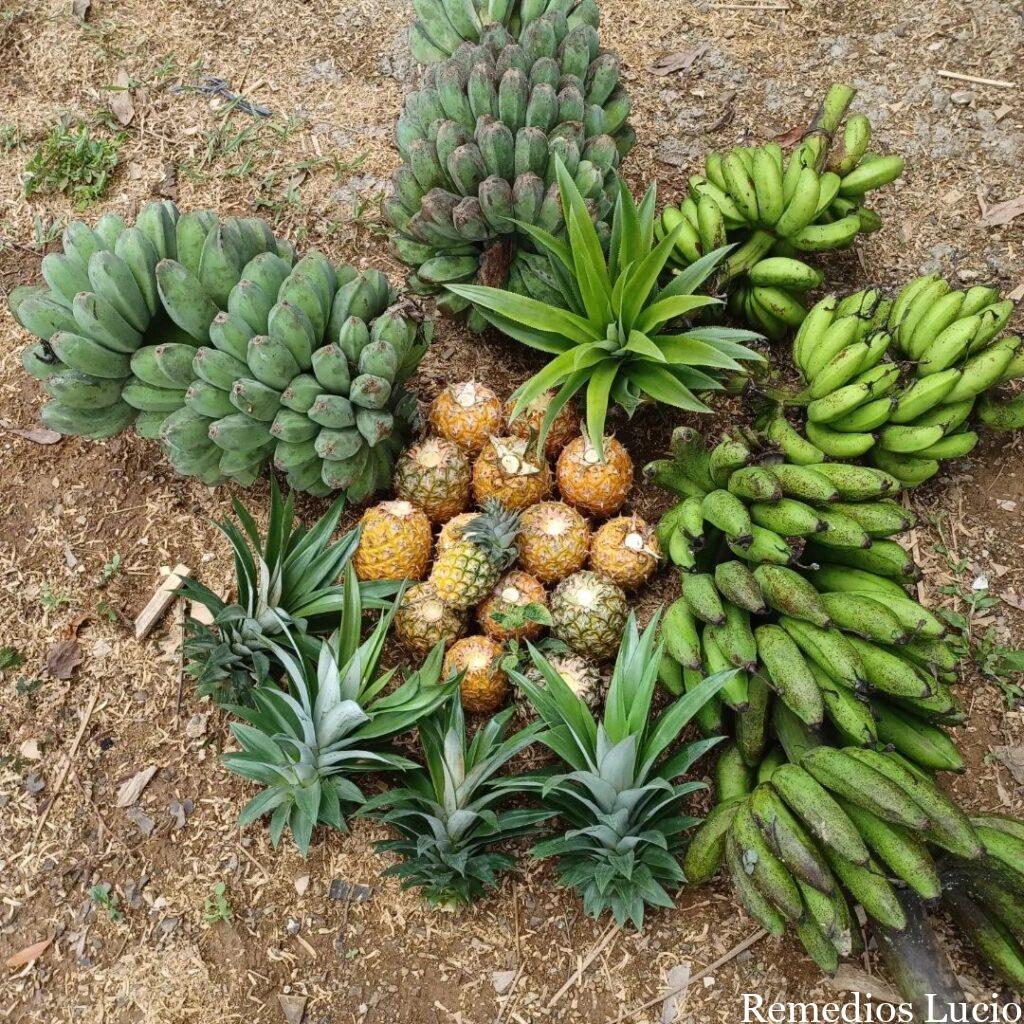The image showcases a vibrant and detailed arrangement of various fruits laid out on a dirt-covered ground. At the center of this arrangement are several pineapples, varying in shades from golden brown to greenish-yellow, and ranging in shape from round to slightly oval. Most of the pineapples have had their leafy tops cut off, with these green leaves arranged around the base of the fruits. Surrounding the pineapples are numerous large bunches of what appear to be bananas and plantains, featuring different shades of green—some a deep green with gray accents, and others a brighter, lighter green. The fruits are artistically arranged to form a star-like pattern, creating an almost shrubbery-like or art piece effect and adding a distinct visual appeal to the earthy setting.